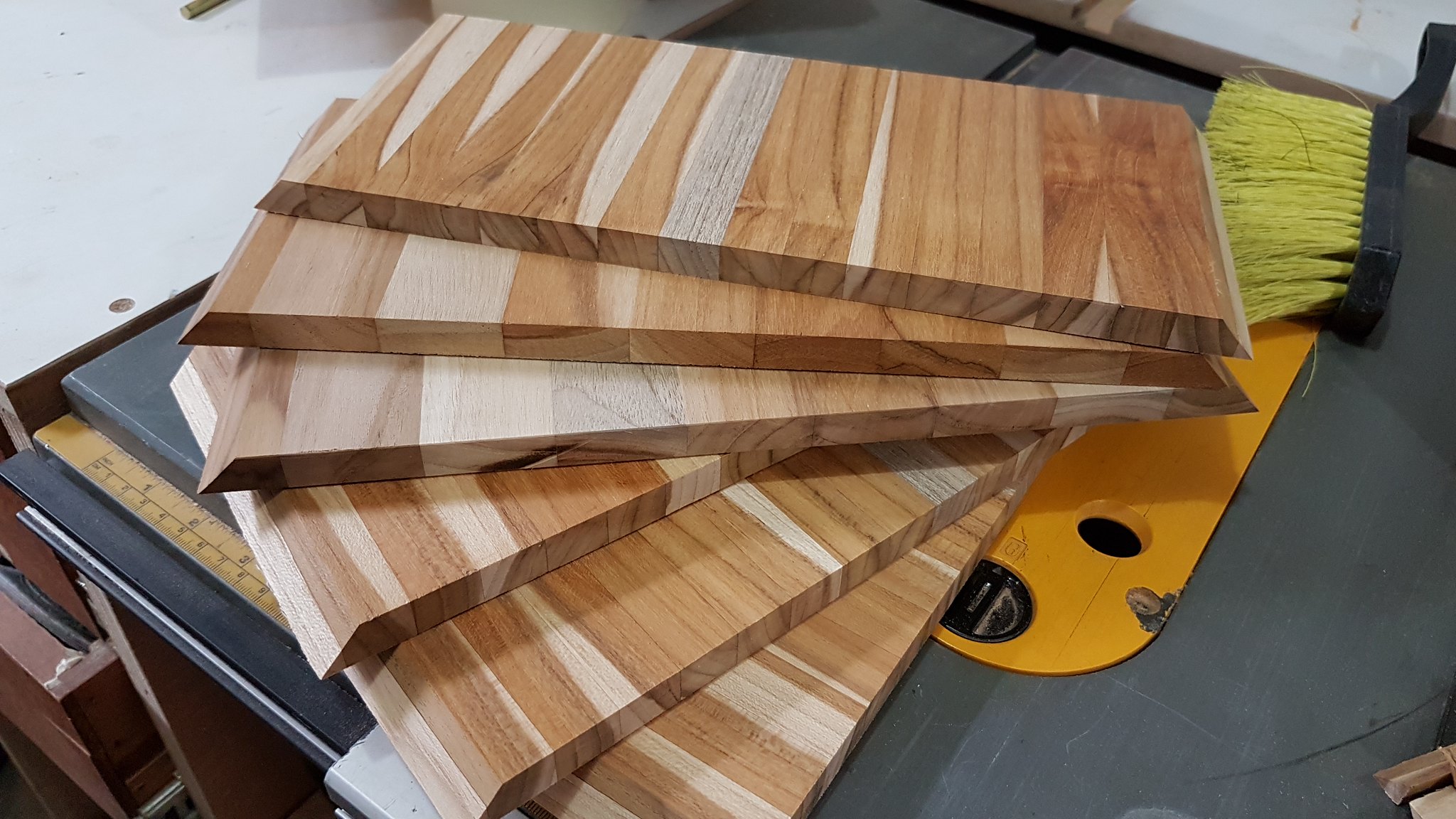The indoor color photograph captures a bird’s-eye view of a table saw situated in a well-lit workshop. On the table saw, six rectangular pieces of laminated wood, showcasing various species and colors, are fanned out to reveal distinct vertical grain patterns. Each piece has slightly beveled edges on the short ends, forming a parabolic profile. In the upper right corner of the table saw, a brush with long yellow bristles points towards the center of the image. The table saw is primarily gray with an orange section in the middle and a yellow ruler featuring black numbers and dashes. The upper left corner of the image shows a white surface, likely a wall or the floor. Despite the numerous woodworking details, the primary focus is on the laminated wood pieces, presented like a hand of playing cards. The image is clear and sharp, emphasizing the textures and contrasting wood tones without any text or print visible.